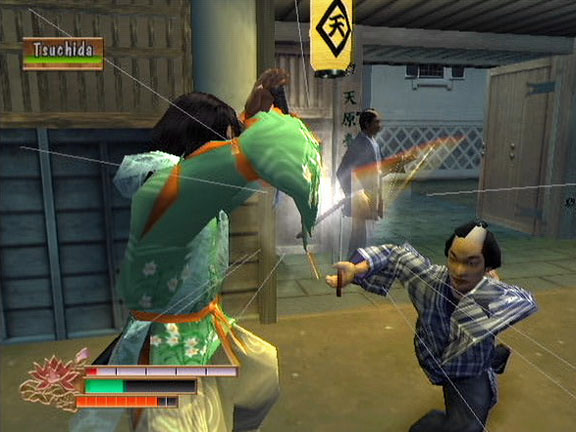This detailed image captures a scene from a retro Japanese video game, reminiscent of the PlayStation 2 era, approximately 20 years ago. The setting appears to be a kite shop with an intricately designed Japanese sign and colorful triangular decorations. The focal point of the image is a woman in a blue dress standing by the door, while in the background, another figure is suspended at an angle from wires, adding to the scene's dynamic nature. 

On the left, large metal doors frame the scene, and at the bottom, health and energy bars track the progress of a combat encounter. The main gameplay action involves two martial arts fighters: one, a virtually miniature fighter in a green flowing shirt with a bow, identified as Tsushida, and another with a traditional samurai hairstyle, possibly wielding a katana, although his body is contorted in an unusual manner. Another potential enemy looms in the background, adding to the anticipation of the battle. The detailing and setup suggest the game's strategic complexity and rich cultural inspiration.